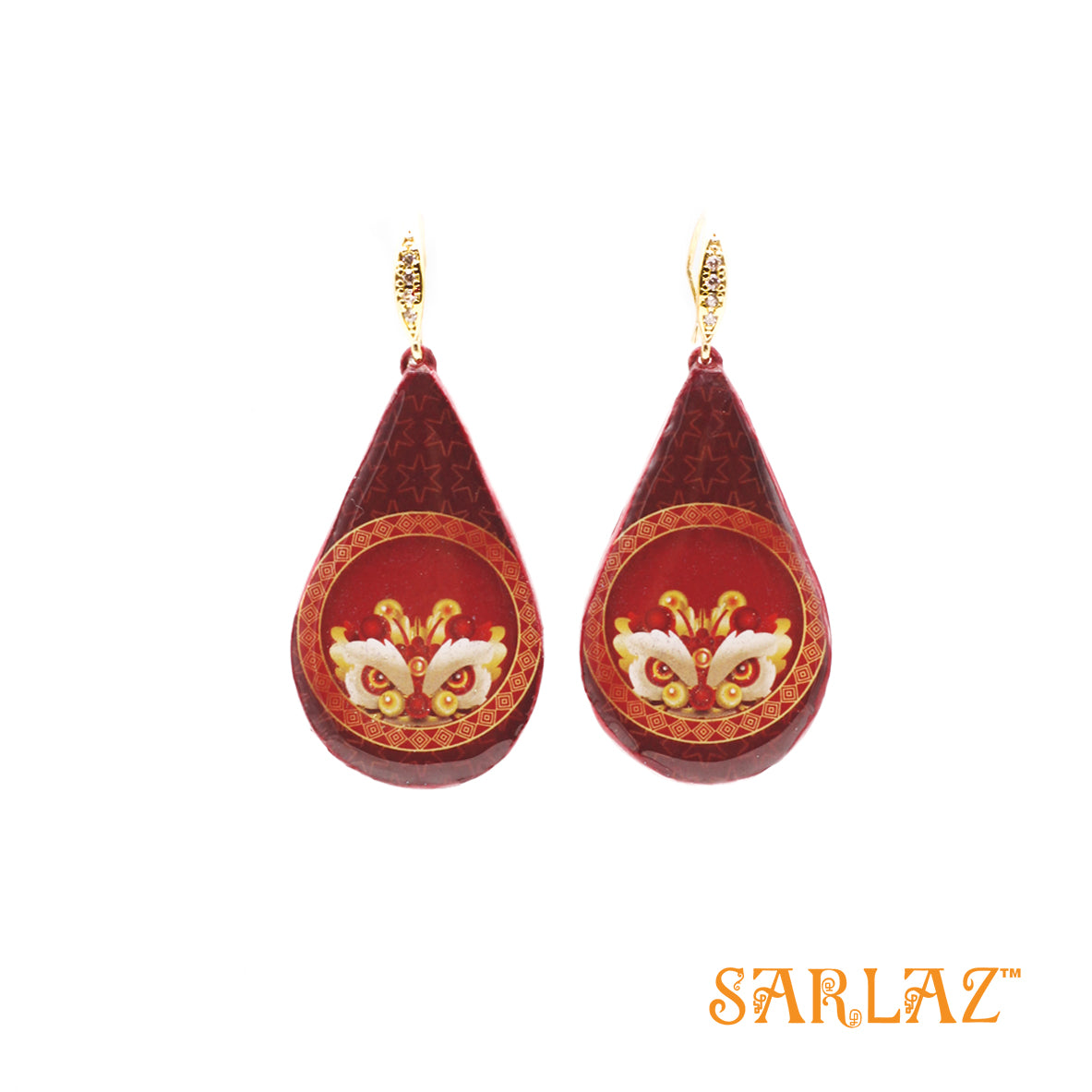The image showcases a pair of teardrop-shaped earrings adorned with intricate designs, set against a blank white background. The earrings hang from golden or brass fittings. The upper part of each earring is dark red, featuring a pattern of stars, while the lower part is a circle encompassing a detailed design that appears to depict an owl-like creature. This creature has red eyes with white centers, yellow and red antennas, and two yellow marks near its nose. Additionally, golden orbs and red orbs can be seen above the owl's head. The bottom edges of the earrings display a triangular design. At the bottom right corner of the image, there's orange text that reads "S-A-R-L-A-Z" with a trademark (TM) symbol next to it.